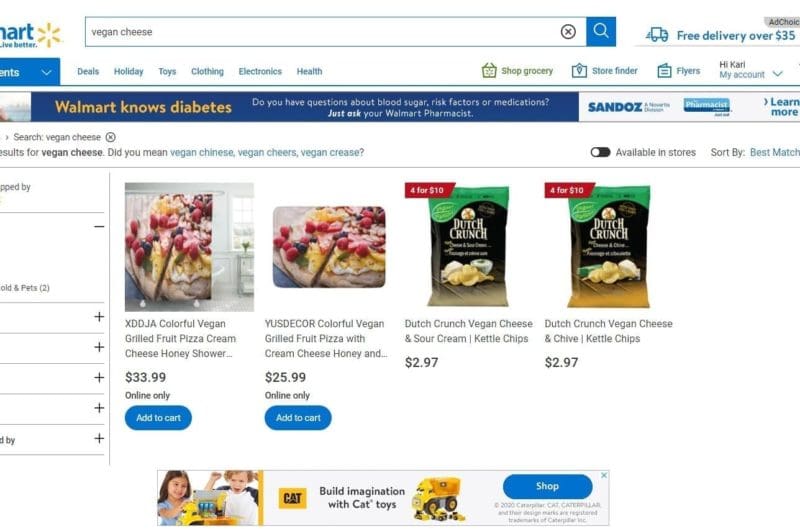The image appears to be a screenshot of a Wal-Mart online shopping interface featuring various sections and promotional information. 

On the upper left, part of the familiar "Wal-Mart" logo along with its iconic yellow sunburst symbol is visible. Positioned centrally on the interface, a blue-outlined rectangle prominently displays the text “vegan cheese,” accompanied by a circle with an X on its left side and a blue square with a magnifying glass icon, possibly indicating a search function.

A truck image with the text “free delivery over $35” is also present, suggesting a delivery promotion. Below this, partially visible, is a blue rectangle with a downward-pointing arrow and some indecipherable text.

A depiction of a bag with the text “shop grocery” and an icon resembling a shield with a map, labeled “store finder,” are also visible. Near these icons is an image of a piece of paper labeled “flyers” and the text “hi, Carl,” alongside a down-pointing arrow, likely relating to user account details.

A blue rectangle features the text “Wal-Mart knows diabetes” in yellow, with supplementary information in white text below. Adjacent is a gray-outlined rectangle with the text “sandos.” Another blue rectangle, transitioning from light blue to dark blue, contains a right-pointing arrow and the phrase “learn more.”

Below these sections are images of various food items, including what seem to be two pizzas and two kinds of chips. These items are labeled with their prices: $33.99 and $25.99 for the pizzas, with both marked “online only” and accompanied by “add to cart” buttons. The chips are priced at $2.97 each.

To the left of these food images is a rectangle showcasing children playing, followed by a gray area. Further down is a yellow rectangle promoting “cat and build imagination with cat toys,” illustrated with toy images and accompanied by a blue “shop” button and some small, unreadable text below.